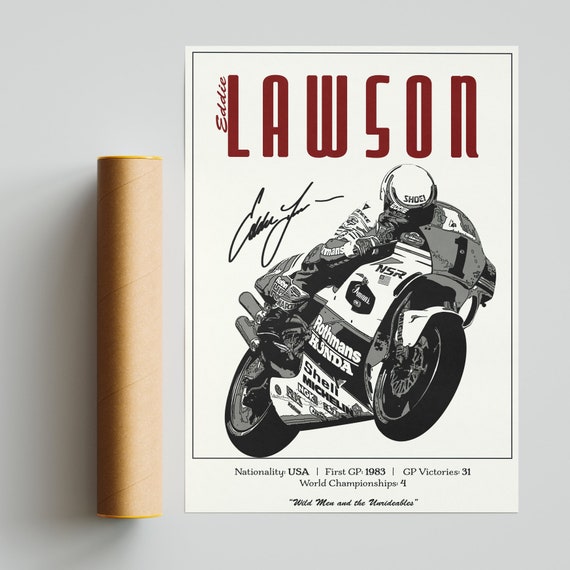In this image, there's a gray background with a poster on the right and a cardboard tube on the left. The poster highlights legendary MotoGP rider Eddie Lawson. At the top of the poster, "LAWSON" is prominently displayed in dark red capital letters, with "Eddie" written smaller and vertically to the left of the 'L'. Below 'Lawson', there is a detailed black-and-white pencil sketch of Eddie Lawson in full gear, riding a motorcycle that tilts slightly to the right. The motorcycle features several sponsor logos, including NSR, Honda, Shell, and Michelin, although some are difficult to make out. The bike, with two blackened tires, displays a number "1" on the front fender, signifying Lawson's ranking. The sketch is signed by Lawson, with the signature located near the helmet. Further details listed at the bottom of the poster include Lawson's nationality (USA), his first GP in 1983, his 31 GP victories, and his four world championships. The poster also features the quote "Wild Men and the Unridables" in quotation marks at the bottom. The tube beside the poster likely serves as packaging for shipping. The sheet of paper, described as somewhat dirty white, further authenticates this collectible item.